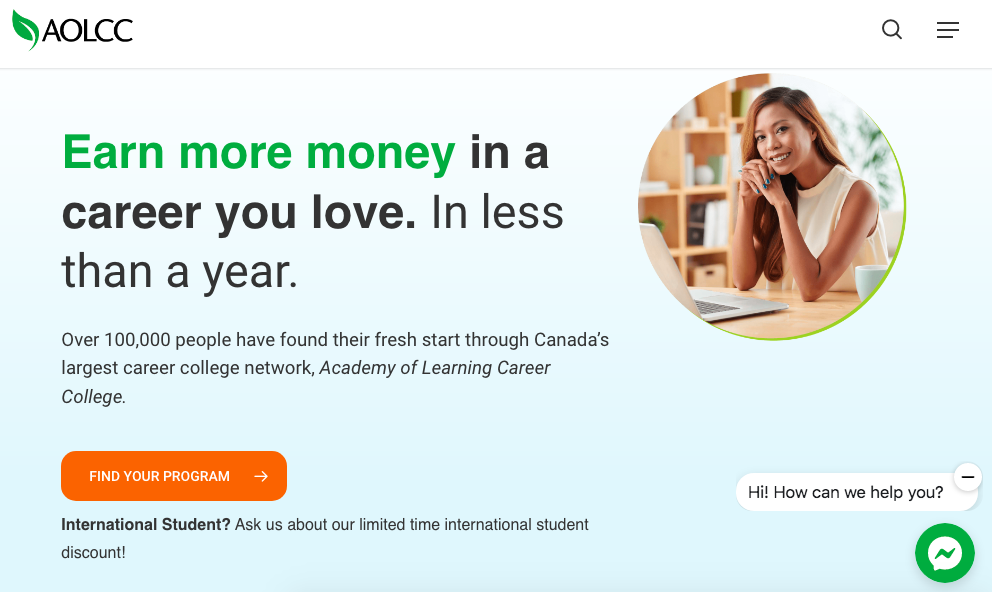On the upper left corner of the image, a small green leaf is present next to the text "A-O-L-C-C." On the right side, there's a magnifying glass icon followed by a stack of three horizontal lines, the last of which is smaller than the two above it. Below this, there's a gray line and under it, a blue rectangle. To the left, in green text, it says "Earn More Money," followed by black text that reads, "in a Career You Love in Less than a Year."

To the right, there's a circular photo of a woman with long hair wearing a white cream-colored shirt. Beneath this photo, the text reads: "Over 100,000 people have found their fresh start through Canada's largest career college network, Academy of Learning Career College." An orange rectangle with rounded edges below this text contains the words "Find Your Program" accompanied by a right-pointing arrow.

Further down, black text says, "International Student? Ask about our limited time international student discount." To the right side of the image, in a white toolbar, it says, "Hi, how can we help you?" Above this text is a circle with a minus sign, and below it is a green circle containing a white speech bubble icon with a slightly crooked end.